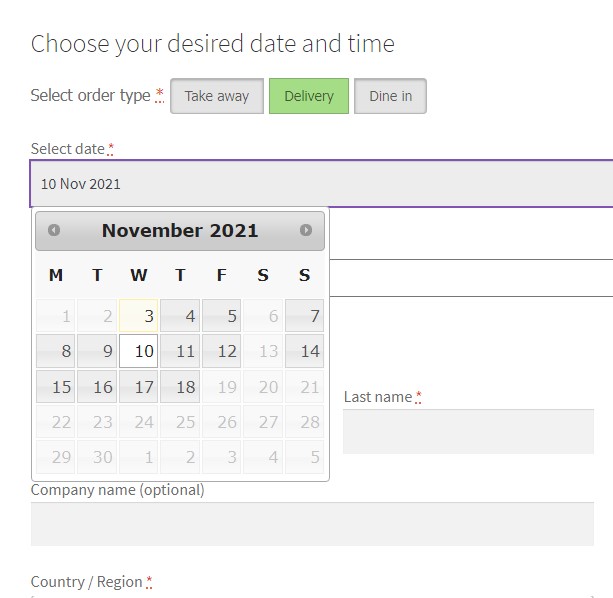This image showcases a webpage for placing a food order. At the top of the page, prominent text invites the user to "Choose your desired date and time." Directly below, it instructs the user to "Select order type," presenting three options in distinct boxes: "Take Away" in a gray box with black letters, "Delivery" in a green box with black letters, and "Dine In" in another gray box with black letters. Moving down the page, the phrase "Select date" is displayed, indicating that the chosen date is November 10, 2021. A calendar interface beneath this shows the month of November 2021, with the 10th highlighted, revealing it to be a Wednesday. The page also contains fields for user information: the top fields are concealed, but one visible field labeled "Last Name" suggests that fields for first and last names are required. Below these fields, another input titled "Company Name (Optional)" is visible. Finally, in the lower left corner, the option to specify "Country/Region" is available.